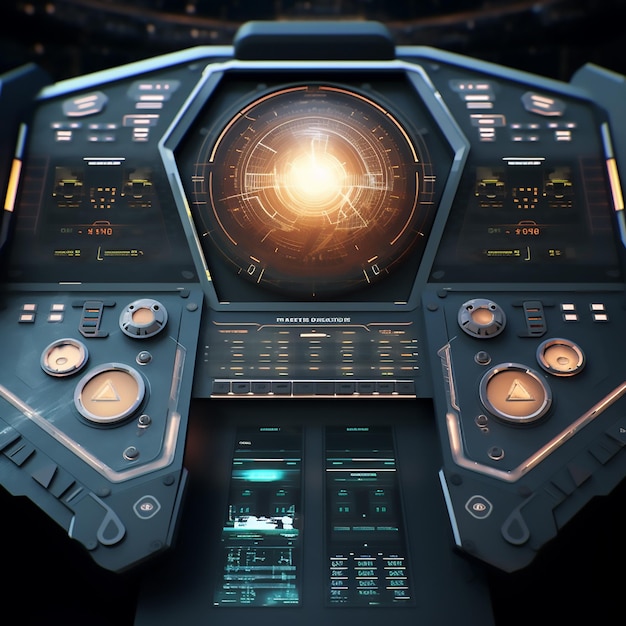The image depicts a highly detailed cockpit or control panel, likely from a spaceship or a futuristic craft, possibly from a fantasy or science fiction context. The cockpit is complex, with a mixture of dark colors and vibrant highlights, primarily in black, gray, orange, and metallic light blue. Dominating the top center is an illuminated screen, resembling an orange sphere with intricate lines and geometric shapes, suggesting advanced technology or an AI interface. Surrounding this central screen is a pentagon frame. Flanking this central setup are symmetrical panels on the left and right, each mirroring the other with numerous dials, buttons, and small screens displaying various readings. At the bottom, there are two vertical panels that resemble cell phones, each filled with controls and data, colored a striking turquoise. Throughout the cockpit, numerous orange buttons and circular dials add contrast against the darker, more subdued background, giving the entire setup a sophisticated yet fictional appearance. The abundance of controls and the futuristic design elements imply this is a crafted image meant to resemble a spaceship's control deck, possibly from a video game or an imaginative artwork.